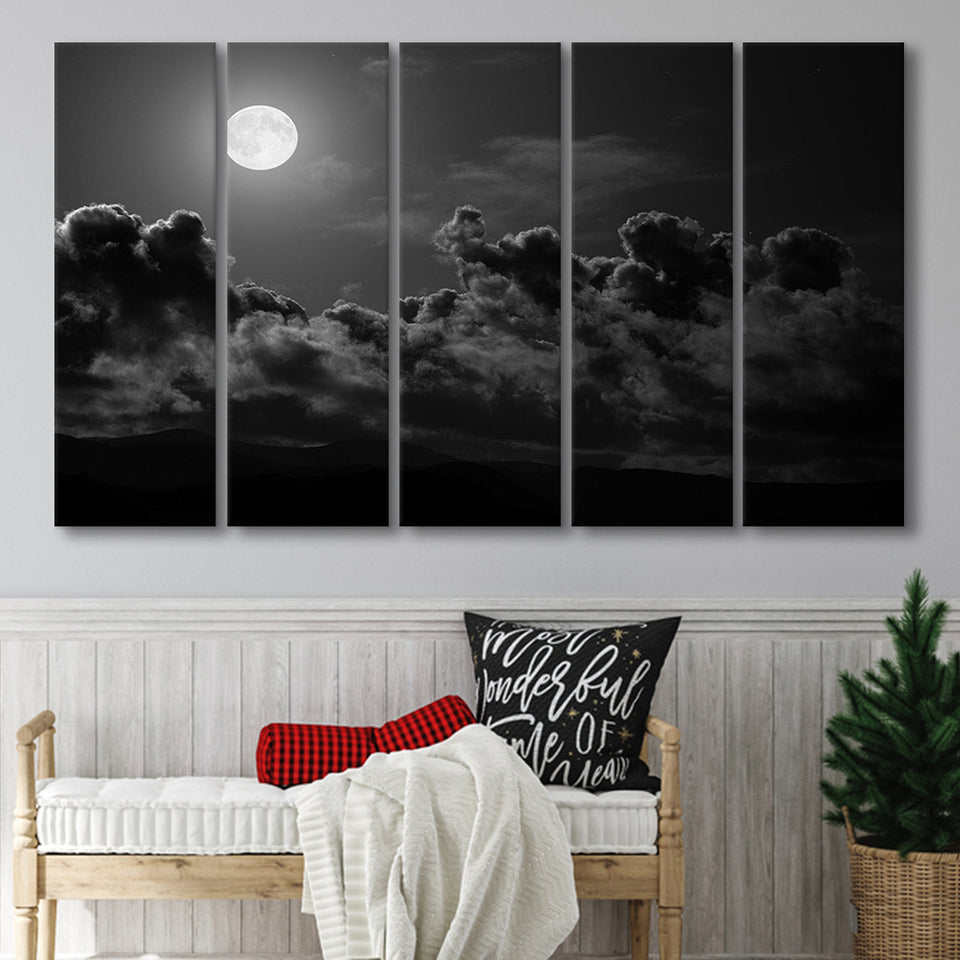The photograph captures a cozy indoor setting within a room of a house. The backdrop features a light gray wall, accented by wooden wainscoting in a similar light gray hue that climbs up about a third of the wall. The two textures are separated by a strip of molding. Dominating the upper portion of the image is a striking five-panel artwork. Each panel, separated by about an inch of wall space, collectively forms a captivating nocturnal scene with a moon glowing amidst rolling clouds in a dark sky.

Beneath this atmospheric artwork is a small wooden bench, complete with a padded cushion and handles on either end. Draped casually over the bench is a white shawl or sweater, adding a touch of softness to the setting. The bench also holds two pillows: one, a small cylindrical pillow in a bold red and black checkered pattern, and the other, a black pillow with the word "wonderful" inscribed. To the right of the bench stands a small wicker basket containing a diminutive evergreen tree, possibly artificial, contributing a natural element to the decor. The overall composition of the photo emphasizes a predominantly monochromatic color scheme punctuated by the vibrant red of the checkered pillow.